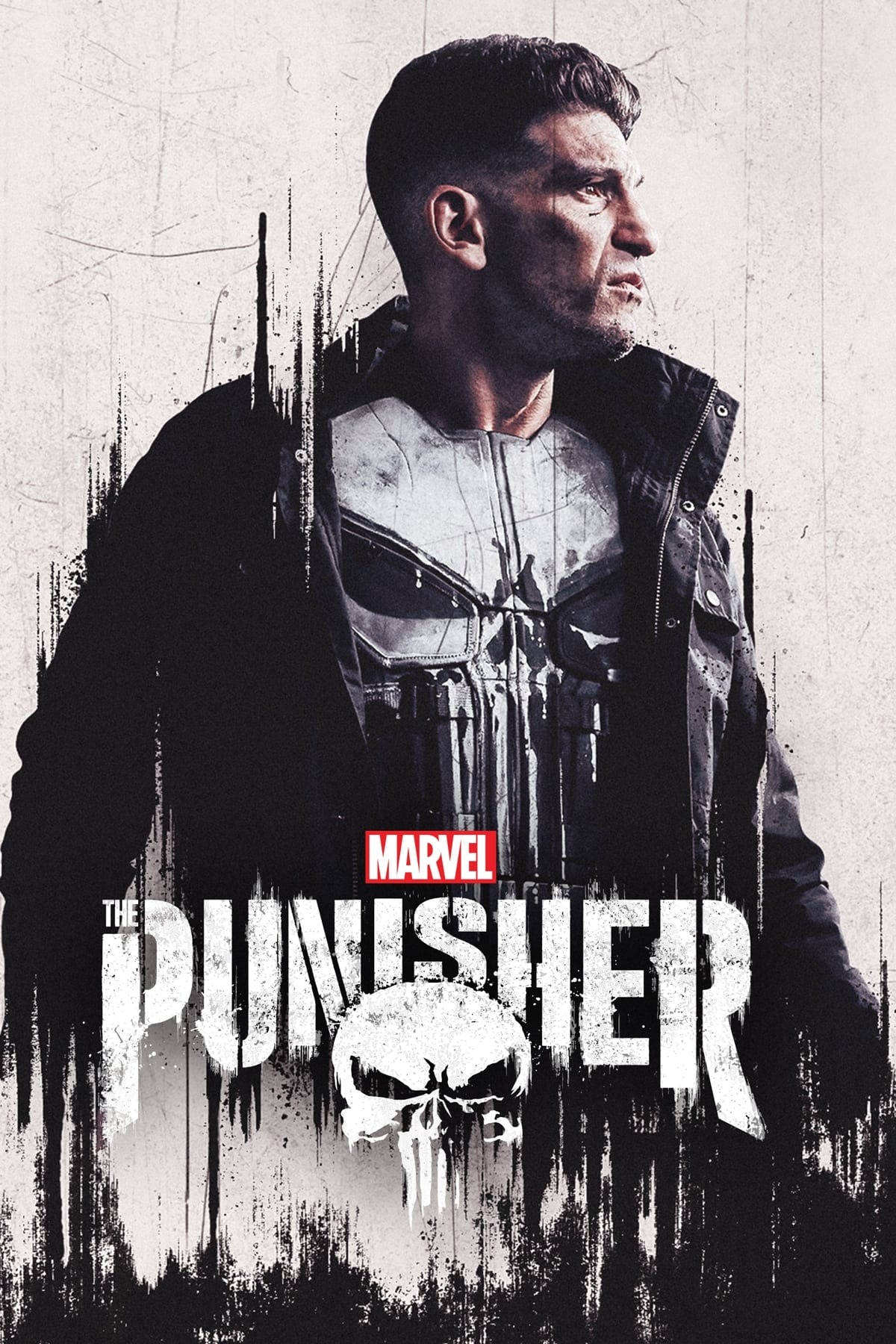The poster for the Marvel series "The Punisher" prominently features actor Jon Bernthal in the titular role. Bernthal, captured in a three-quarter profile with his intense gaze directed to the right, sports a black leather jacket over a black t-shirt emblazoned with a distinct white skull logo, which appears to be melting. His dark, slightly curly hair adds to his intense demeanor. The background of the poster is a gritty, whitish-gray with black splotches and streaks, enhancing the hard-edged aesthetic of the series. The Marvel logo, displayed in white within a red text box, tops the poster, signaling the show's creators. Below Bernthal, in a bold, stencil-style font with a spray-paint look, is the word "Punisher," accompanied by a half-skull insignia between the words, anchoring the graphic intensity of the design.